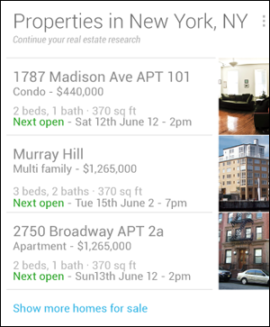The image is a small advertisement on a white background. The majority of the text is in gray, with some highlighted details. 

The heading, in the largest font, reads: "Properties in New York, New York." This is followed by a call to action: "Continue your real estate search and research." 

Three real estate offerings are presented:

1. **1787 Madison Avenue, Apartment 101**:
   - Type: Condo for Sale
   - Price: $440,000
   - Specifications: 2 bedrooms, 1 bathroom, 370 square feet.
   - Next Open House: Saturday, June 12th at 2 p.m.
   - Image: Interior view of the condo.

2. **Murray Hill**:
   - Type: Multifamily
   - Specifications: 3 bedrooms, 2 bathrooms, 370 square feet.
   - Next Open House: Tuesday, June 15th at 7 p.m.
   - Image: Exterior view of the building (Interior not shown).

3. **2750 Broadway, Apartment 2A**:
   - Type: Apartment for Sale
   - Specifications: 2 bedrooms, 1 bathroom, 370 square feet.
   - Next Open House: Sunday, June 13th at 2 p.m.
   - Image: Exterior view of the apartment building.

All properties listed share the improbable feature of measuring 370 square feet, which is unusually small given the number of bedrooms and bathrooms. Additional properties for sale are mentioned, indicating a broader inventory.